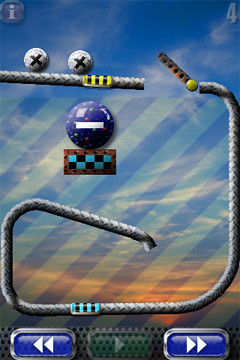The image depicts a screenshot from a mobile puzzle game, characterized by its vertical orientation typical of phone displays. The background showcases a serene blue sky adorned with wispy white clouds and hints of yellow and orange, suggesting a sunrise or sunset. Central to the game, a series of small white balls, each marked with a black X, navigate down a track resembling a metal rope, aimed towards an orange-red, spiral-shaped contraption that appears to be an interactive hinge or swing. Below this, a larger blue ball, speckled with green and pink dots and bearing a white minus sign, rests on a rectangular brick with a distinct turquoise and black checker pattern. The interface includes navigational buttons at the bottom, featuring left and right arrows set against white and blue backgrounds, indicative of player controls.